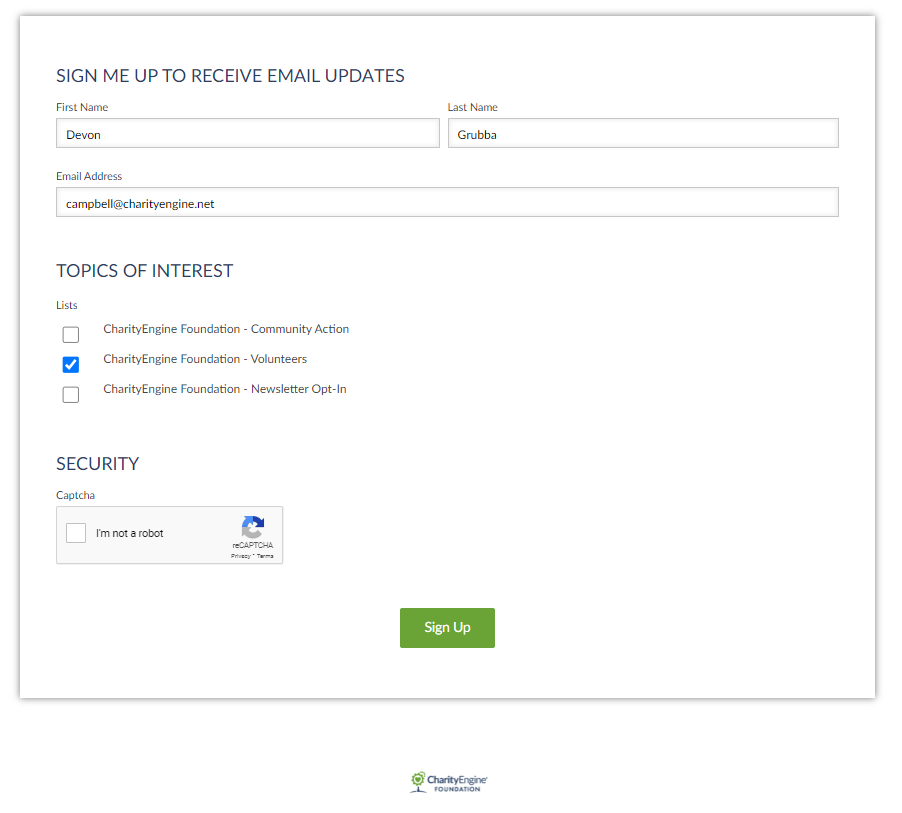The website image depicts a sign-up form bordered in light gray. The form contains a header that instructs users to "Sign me up to receive email updates." Within the form, there are fields for "First Name" and "Last Name," with the example entries "Devon" and "Grubba" respectively positioned side by side.

Below these fields, there is an "Email Address" section filled with the email "Campbell@CharityEngine.net." Farther down, a section titled "TOPICS OF INTEREST" in gray, uppercase letters presents selectable options, each accompanied by a square checkbox. The options include:
1. Charity Engine Foundation Community Action
2. Charity Engine Foundation Volunteers
3. Charity Engine Foundation Newsletter Opt-in

The "Charity Engine Foundation Volunteers" option is marked with a blue box containing a white checkmark, indicating selection.

At the bottom of the form is a security verification section labeled "CAPTCHA." This section features text stating "I'm not a robot" next to a square checkbox that users must click on for verification. Additionally, the CAPTCHA includes a gray-blue circular arrow icon, typically used to refresh the CAPTCHA challenge.